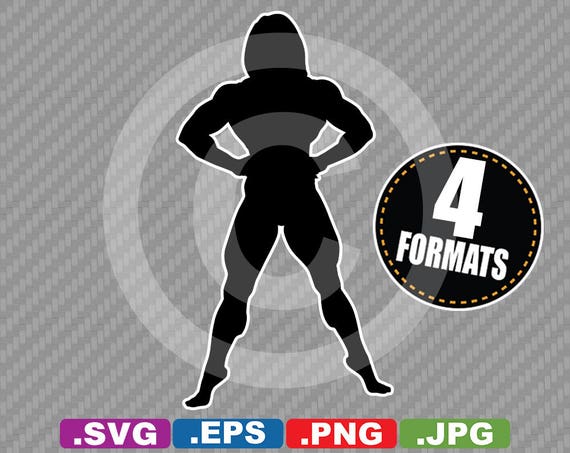The image features a detailed and dynamic graphic design set against a gray background with lighter and darker gray diagonal stripes. At the center of the image, there is a bullseye-like design that includes a white letter "C" in the middle of a series of concentric circles, with the outermost circle being lighter than the background stripes.

Dominating the center of the graphic is the silhouette of a person who appears to be a bodybuilder or superhero. This muscular figure, which could be either male or female, stands in an assertive pose with feet apart and hands on their hips, elbows bent outward. The silhouette is primarily black, segmented by alternating gray areas from the head down through the wrists, waist, knees, and ankles, creating a striking contrast with the white outline that borders the figure. Noticeably, the figure stands on tiptoes, and the flowing hair suggests a powerful presence.

To the right of the figure, there is a prominent black circle with a white border and yellow stitched edges. In the center of this circle, the text "Four Formats" is displayed in white letters. Below this circle, at the bottom part of the image, four colored boxes list different file formats with their respective extensions: a purple box with "SVG," a blue box with "EPS," a red box with "PNG," and a green box with "JPG." 

The overall art style combines elements of superhero aesthetic with a sleek, modern background, making it both visually striking and informative.